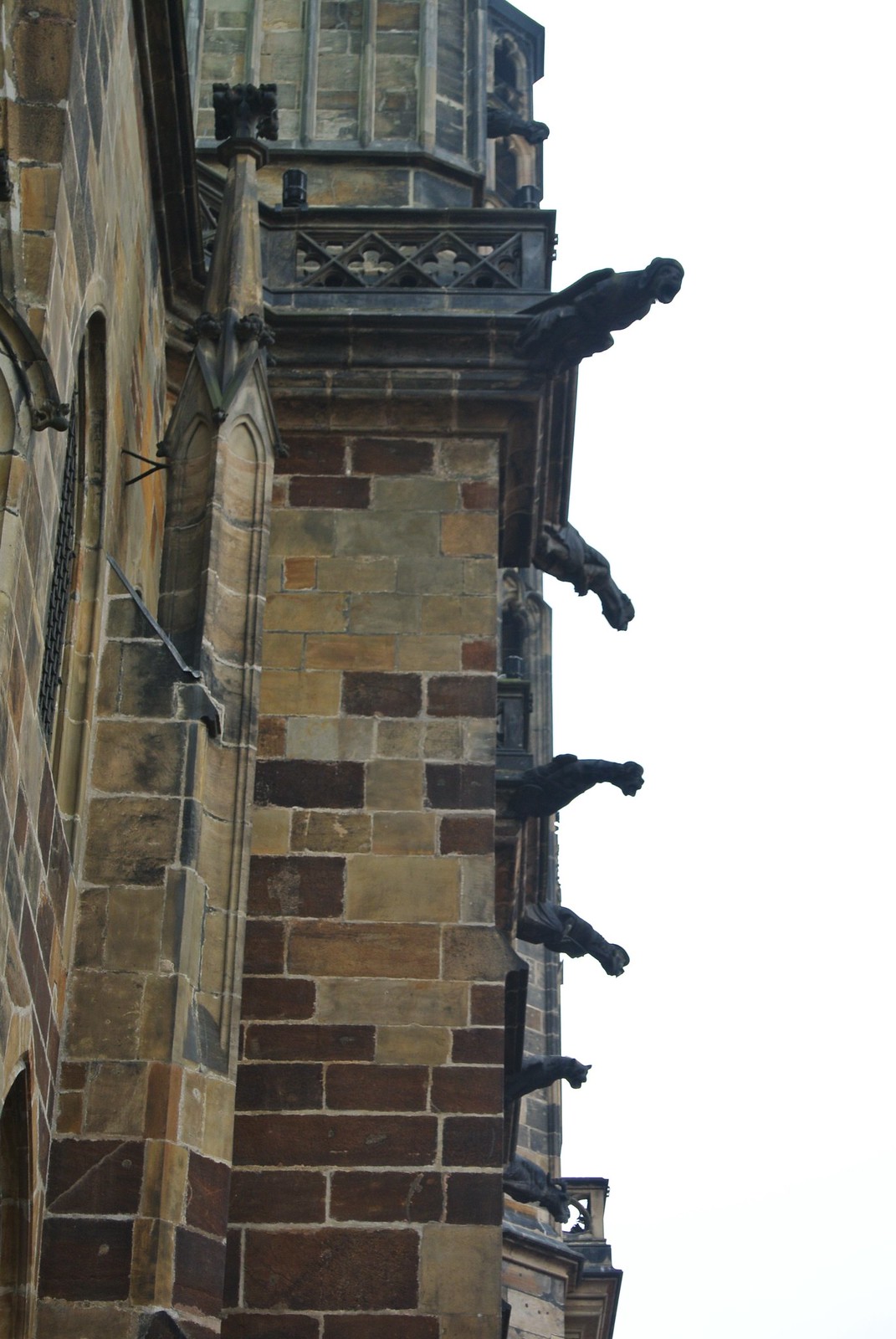The photograph captures a towering, multi-hued brick structure, likely a cathedral or castle, bathed in a white overcast sky. It presents a medieval English design with dark brown, light brown, gray, and tan bricks forming an intricate exterior. Dominating the left side of the image, the edifice features a sequence of six small, dark gargoyles protruding along the right edge of the structure, typical of Gothic architecture from the Middle Ages. Below a dark wooden railing adorned with a diamond pattern—reminiscent of lighthouse top designs—rests an area echoing cathedral grandeur. High on the left wall, an arched, dome-shaped window punctuates the brick expanse, adding to the historic ambiance. The building’s protruding sections and detailed masonry augment the photograph’s depth, bringing to life the ancient grandeur and architectural finesse of this majestic structure.